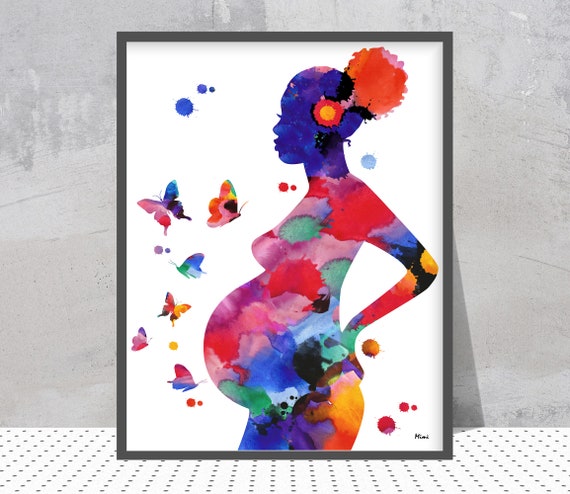The image depicts a vibrant, framed artwork that showcases an abstract, multicolored silhouette of a pregnant woman. The artwork is set on a black-framed white canvas, with a light gray concrete wall serving as the background and a white polka-dot covered surface below. The woman is rendered in an array of watercolor hues, including red, orange, yellow, green, light blue, dark blue, and purple, giving her a tie-dyed appearance. She stands in a side profile, with her hair styled in a bun and adorned with a red and yellow flower, blue earrings, and a fluffy pink and red bow. She wears a colorful dress, and several vibrant butterflies in shades of pink, blue, orange, green, and yellow flutter around her prominent belly. Her hands rest on her back and hips, adding to the dynamic and creative expression of the painting. Paint splatters accentuate the lively scene, and a signature is visible in the bottom right corner.